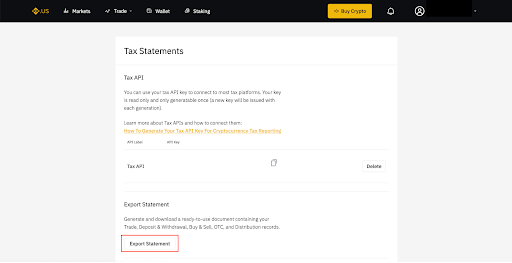The screenshot features a user interface design with a light gray background. At the very top horizontally, there is a black rectangular strip with small print on it. Within this strip, there's a yellow-gold logo accompanied by a name, flanked by three white options. Towards the right side of this strip, there is an orange-gold button, an alarm icon, and a profile circle.

Below the black strip, the background remains light gray, and centrally located is a prominent white rectangle. In the upper left-hand corner of this rectangle, the text "Tax Statements" is displayed in black. A few lines below, there is a horizontal light blue line extending across the page.

Following this line, the content is divided into three sections, each separated by additional light blue lines:

1. **Tax API**: This section includes a paragraph of text, a single sentence, and a gold hyperlink.
2. **Tax API (Continued)**: Positioned to the right within this section is an "Explore" button.
3. **Export Statement**: This section contains two lines of black text, and below this text, there is a rectangular button outlined in red with the label "Export Statement."

The organized layout maintains clarity and accessibility, highlighting key actions and information.